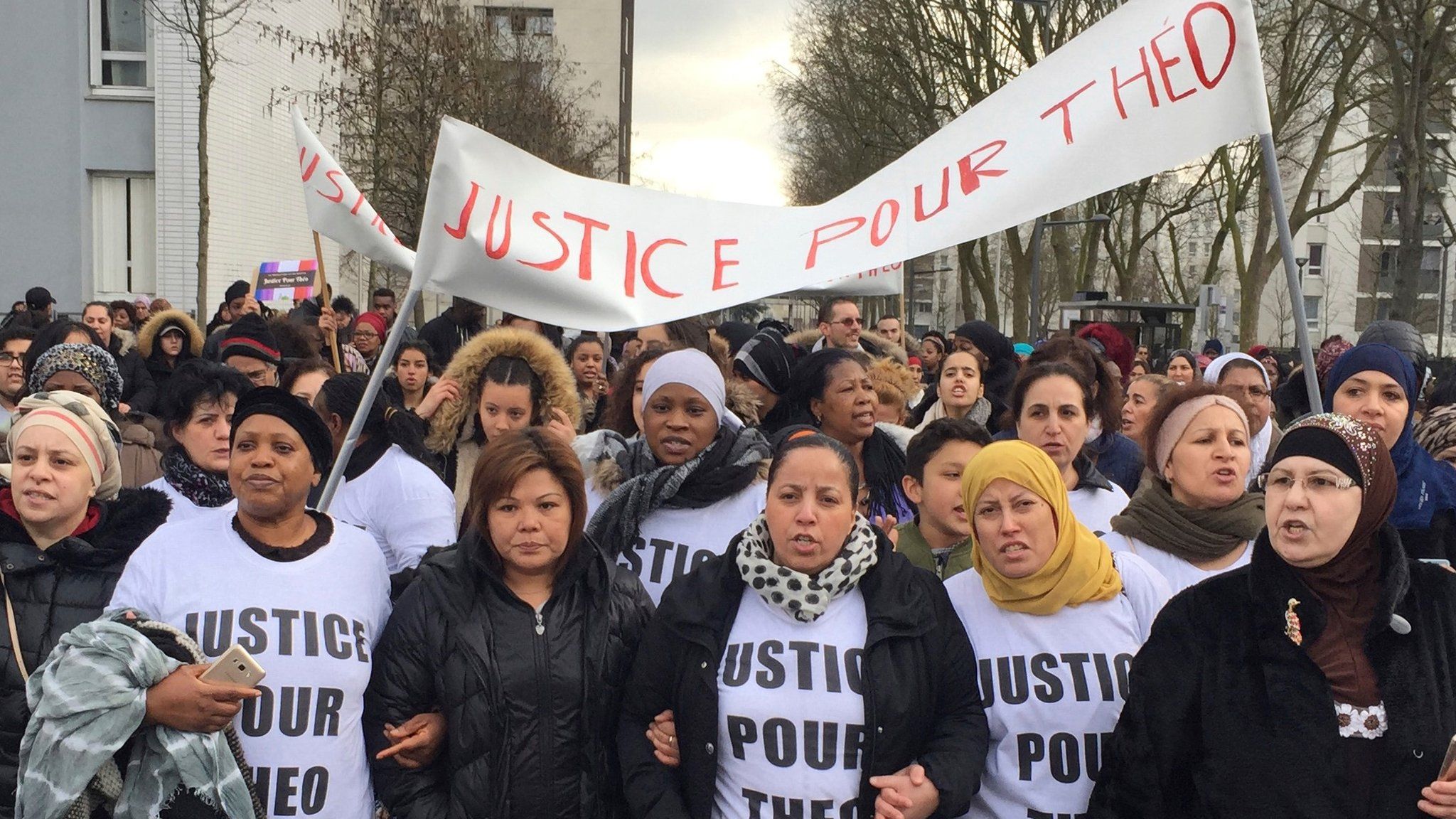The image is a color photograph in landscape orientation, capturing a detailed scene of a demonstration march taking place in a city street. The crowd, composed predominantly of women and young teens, many of whom appear to be of Islamic faith due to their diverse head coverings, spans the entire width of the image near the bottom. They are united under a large overhead banner that is white with red handwriting reading, "Justice Poor Theo." The same message, "Justice Poor Theo," is echoed on the numerous white t-shirts worn by the demonstrators, written in black text. 

Several head coverings of various colors, including black, white, gold, and blue, are visible among the protestors, with some wearing black jackets and others having fuzzy hoods. In addition to the main banner, a person in the back left of the crowd is noticeably holding a red, white, and blue sign. The procession takes place amidst a town or city setting, with white and gray buildings and trees in the background, suggesting a European locale. The women at the forefront have their arms interlocked, emphasizing solidarity and unity in their cause for justice for Theo. The image, rendered in a photographic representational realism style, vividly captures the demonstration's dynamic and the protestors' strong sense of purpose.